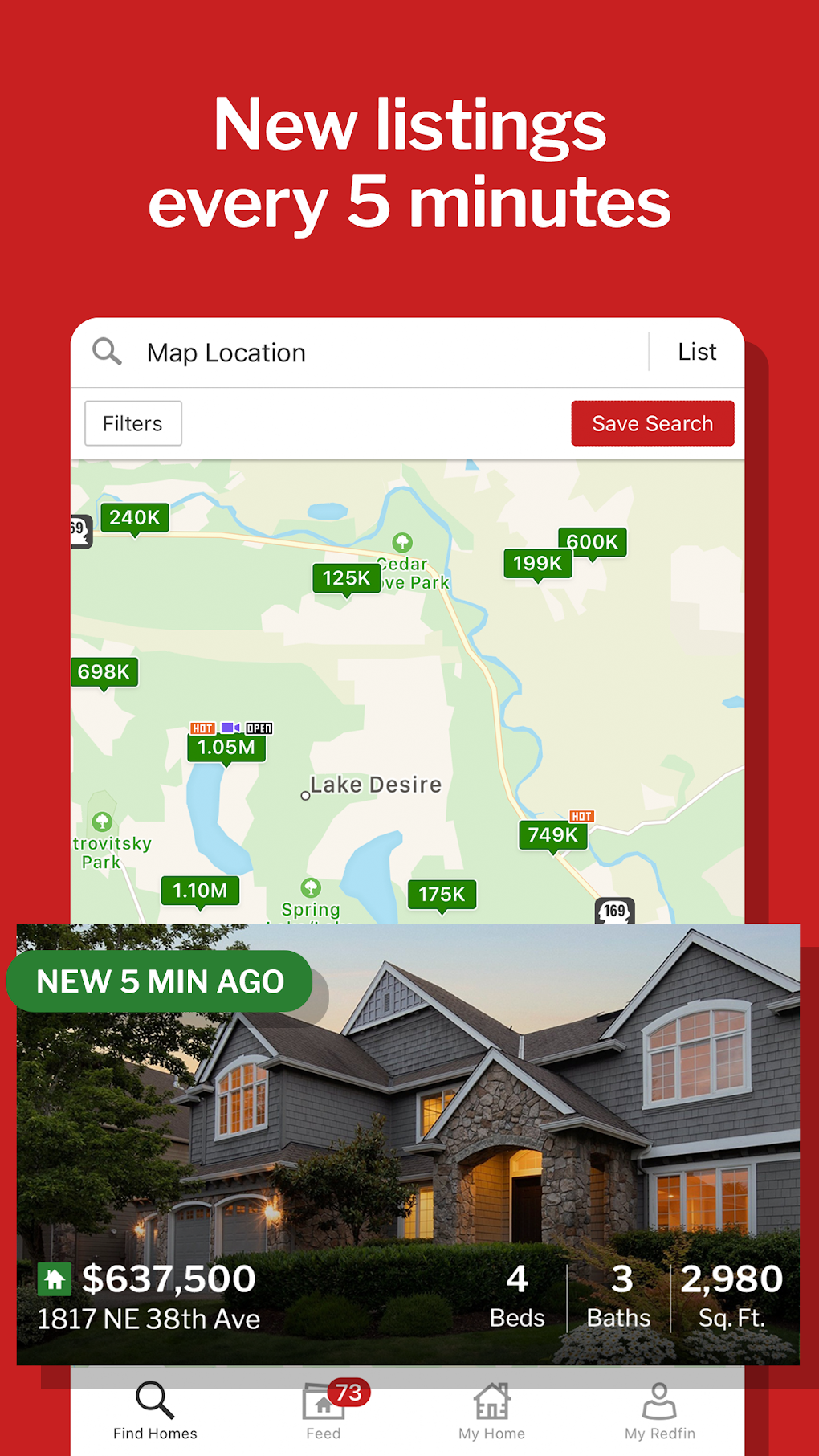This image is a promotional graphic for a real estate company, highlighting new listings available every five minutes. The background is vibrant red, with text in bold white letters prominently stating, "New listings every five minutes." 

At the center of the image, there's a smartphone-shaped element depicting an interactive map interface. At the top of the map, users can see a search icon labeled "Map Location" adjacent to a "List" option in the right corner. Just below, there are interactive buttons: a "Filters" option encapsulated in a white box, and a "Save Search" button in a red box.

The map displays various properties using green square pins, each indicating property prices. The map illustrates a geographic area featuring two lakes, surrounding land, and a meandering river. 

Below this interactive map, there's a thumbnail image of a newly listed gray house, with a timestamp indicating it was listed "New five minutes ago." The image captures the house’s exterior during twilight, with the setting sun illuminating the sky. The house features characteristic A-frame architecture above each window, warm interior lights shining through, a lush green bush around it, and a tree near the right side of the garage.

Key listing details are clearly provided: 
- Address: 1817 Northeast 38th Avenue
- Price: $637,500
- Bedrooms: 4
- Bathrooms: 3
- Total Square Footage: 2,980 square feet

At the bottom of the smartphone interface, users can see a navigation menu with icons labeled for "Phone," "My Profile," "My Home," "Feed," and "Find Homes."